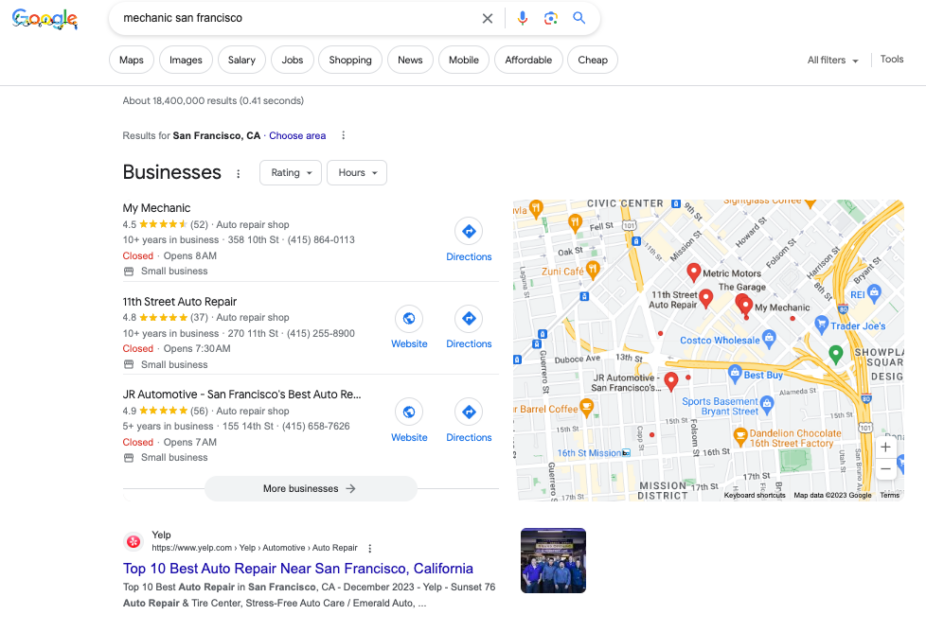This screenshot captures a Google search results page with a festive touch. The background is predominantly white, providing a clean canvas for the content. At the top left, the colorful Google logo is decked out with multicolored Christmas lights strung throughout, adding a cheerful holiday vibe.

Next to the logo, the search bar, in a white elongated pill shape with a subtle light grey shadow, displays the search query "Mechanic San Francisco" in black text.

Below the search bar, a row of white pill-shaped buttons with thin light grey outlines and black text provide quick access to filtered search options like Maps, Images, Salary, Jobs, Shopping, News, Mobile, Affordable, and Cheap. A gap to the right of these buttons leads to grey text reading "All Filters," accompanied by a grey downward-facing triangle, a thin light grey separator line, and the word "Tools."

A thin light grey line separates the header from the main body of the page, also set against a white background. At the top left of the main body, light grey text indicates "About 18 million of 400,000 results (0.41 seconds)." This is followed by black bolded text "Results for San Francisco CA," a medium grey dot, and purple text saying "Choose Area." To the right, three medium grey dots are stacked vertically.

The left side of the screen displays the bolded black heading "Businesses," followed by three grey dots. Two white rectangular buttons with rounded corners and thin light grey outlines are positioned to the right of these dots, labeled "Rating" and "Hours" in dark grey text with corresponding downward-facing triangles.

Beneath this heading are the individual listings. On the left, medium-sized black text identifies a business named "My Mechanic." To the right of the listings is a large map featuring beige and grey land areas, with white and yellow roads. The map is peppered with a multitude of blue and red pins indicating various locations.